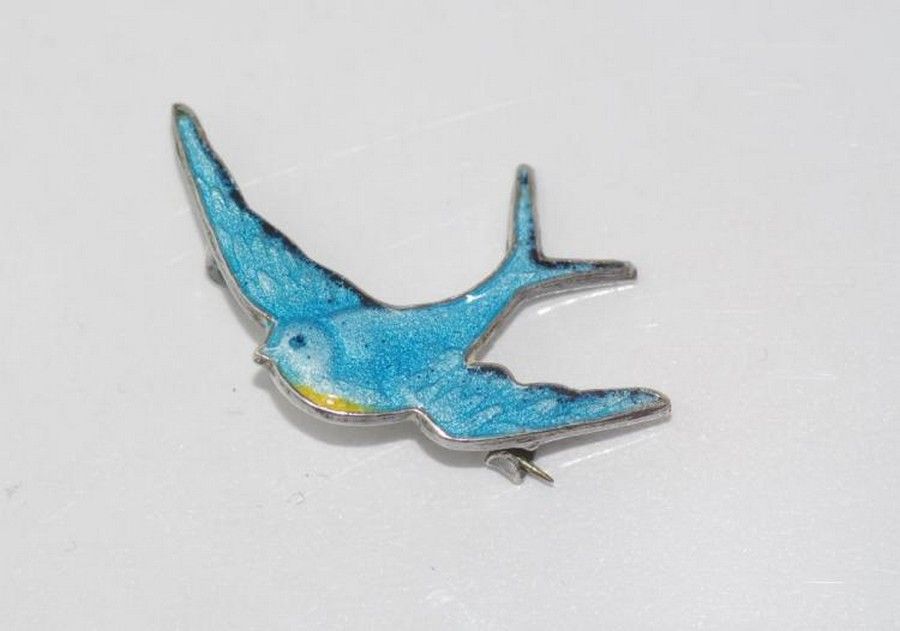The image is a close-up photograph of a decorative pin depicting a bright blue bird, occupying approximately 75% of the frame, and set against a white background. The bird, crafted from a glossy, translucent material such as resin or glass, features a yellow underbelly and a small dark eye. It appears to be in flight, with its v-shaped tail and wings spread out, the latter shaded with black edges that catch highlights from the surrounding light. The speckled blue body of the bird exhibits a slight bubble-like texture due to the glaze. The pin has a silver backing, parts of which are visible under the wings and at the tail, indicating where it would attach to a cloth. The overall composition and close details, like the reflection of light on the wings, contribute to the intricate and vibrant depiction of the bird.